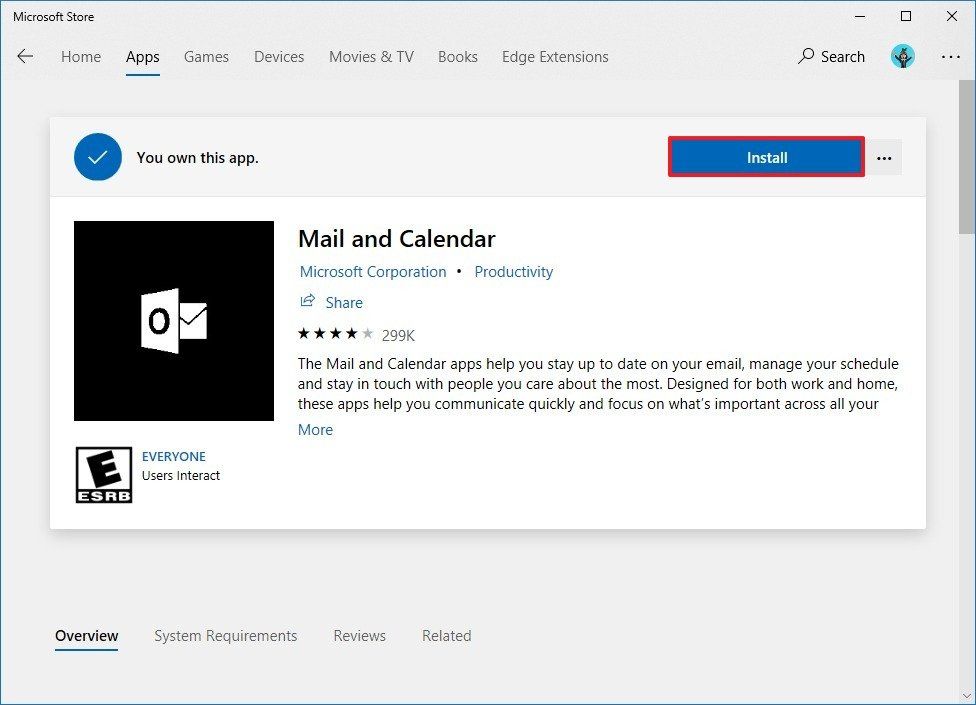Screenshot of the Microsoft Store webpage featuring the Mail and Calendar app:

The screenshot showcases the Microsoft Store interface with a grey background. At the top left, the words "Microsoft Store" are clearly visible. On the right side of this header, there are three buttons: a minus sign, a square for resizing, and an X for closing the window.

Beneath the header, a back arrow points to the left. The navigation menu presents several options: Home, Apps (which is highlighted in dark ink with an underline), Games, Devices, Movies & TV, Books, and Edge Extensions. On the far right, there is a search icon accompanied by the word "Search," a small circle containing an animated person, and a three-dot menu.

Below the navigation menu, there is a rectangular inset box. Its top bar reads "You own this app," featuring a blue circle with a checkmark inside. To the right, there is a blue button labeled "Install" with a red border, and a square containing three dots.

The main section of this inset box displays details about the app "Mail and Calendar" by Microsoft Corporation, categorized under Productivity. An icon with a white envelope on a black background represents the app. Next to it, an "E" for Everyone rating by ESRB, along with the label "Users Interact."

Further details include a share symbol, a 4-star rating based on 299,000 reviews, and a brief description: "The Mail and Calendar apps help you stay up to date on your email, manage your schedule, and stay in touch with people you care about the most. Designed for both work and home, these apps help you communicate quickly and focus on what's important across all your..." The description is truncated, with a clickable "More" link in blue to read further.

At the bottom of the screenshot, on the grey background, navigational options include Overview (highlighted), System Requirements, Reviews, and Related.